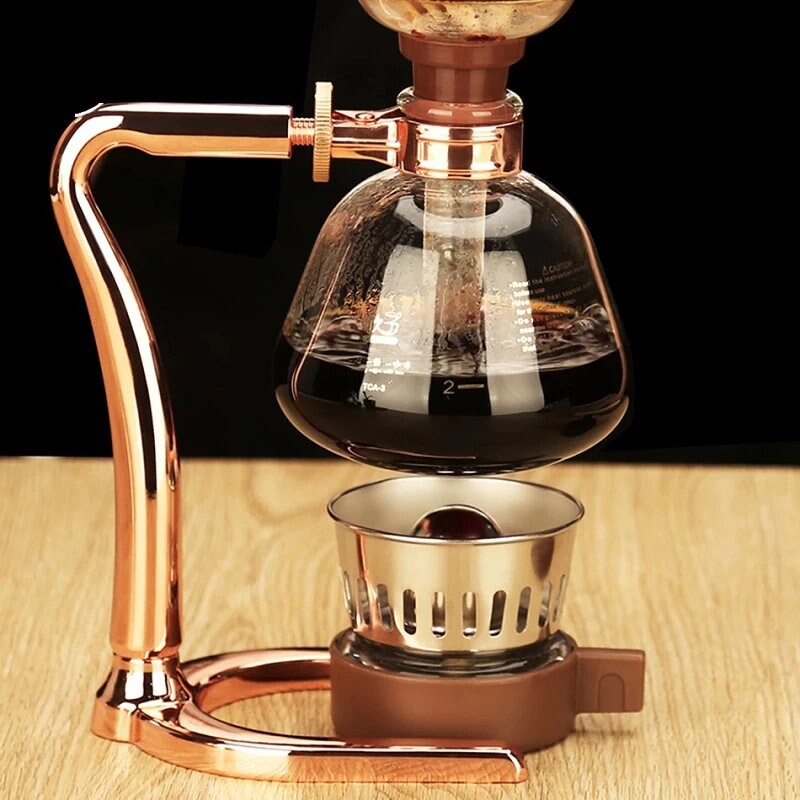The photograph captures an intricate, boutique coffee maker that resembles a scientific apparatus. This elegant machine, possibly made of copper or a shiny metal like chrome or rose gold, sits on a white wood-grained table against a stark, black background. The setup includes a burner reminiscent of a Bunsen burner at its base, surrounded by a round metallic stand. Above the burner, a glass beaker containing a dark brown liquid, likely coffee, is suspended by a copper arm extending from the base. This glass vessel features measurement markings and a central tube, possibly for steam release, and a plastic component protruding from the top. The beaker's liquid is about halfway full, and while the heater appears off, the device gives the impression of sophisticated, methodical operation akin to a chemistry lab.